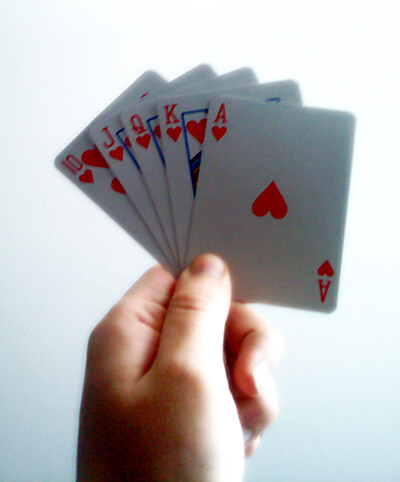In the image, a neatly manicured white hand is holding a fanned-out set of five playing cards. The hand, characterized by short, round nails, grips the cards delicately between the thumb and index finger, specifically at the bottom left corners. The cards displayed are all from the suit of hearts and are arranged in a spread, revealing the top left of each card. From left to right, the cards are: ten of hearts, jack of hearts, queen of hearts, king of hearts, and ace of hearts. The ace of hearts is fully visible at the front of the spread, showcasing its entirety, while the other cards are partially obscured. The background of the image transitions smoothly from white at the top to a light blue at the bottom, giving the scene a serene and clean aesthetic.